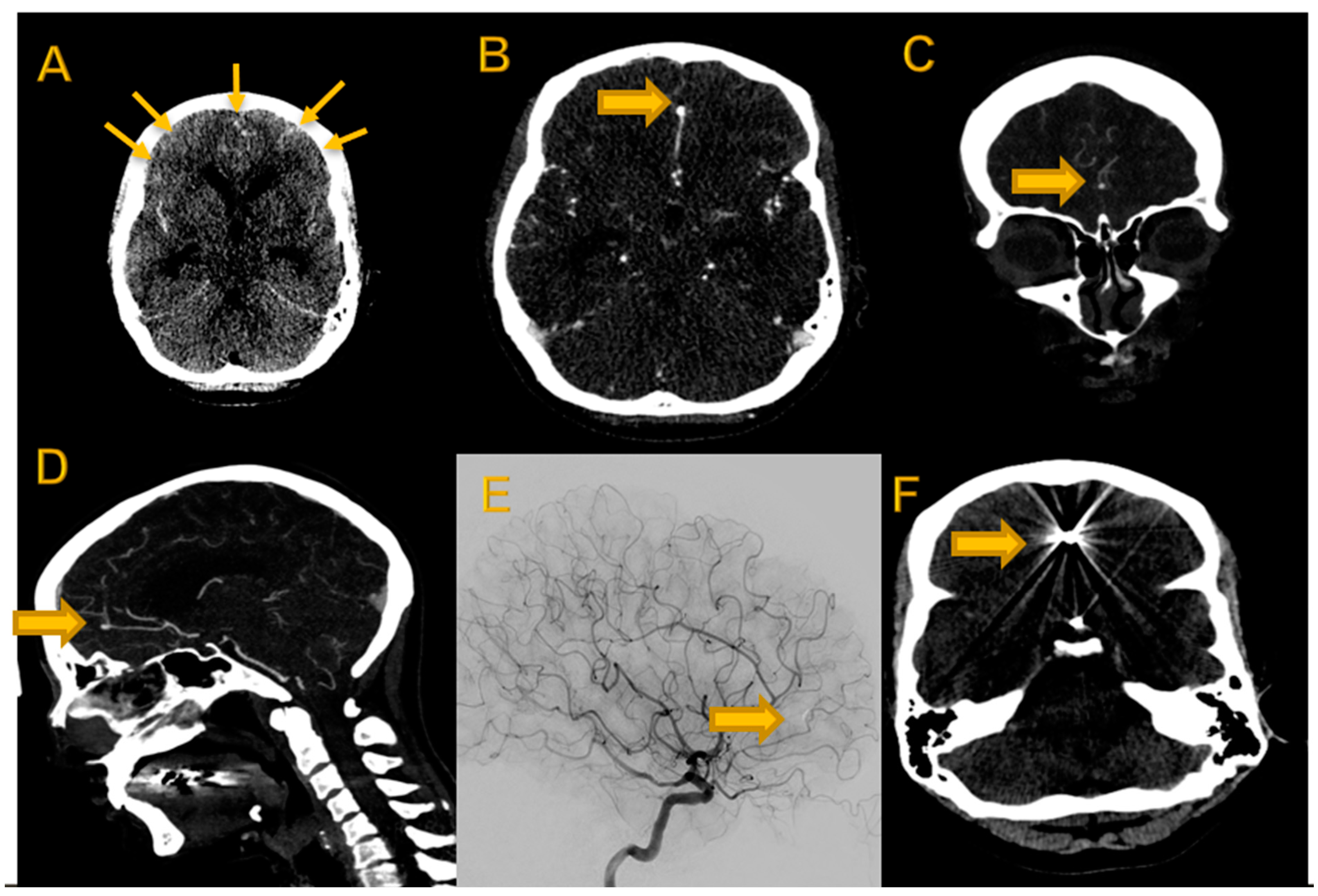This black and white composite image features six different medical images of a brain and skull, labeled A through F. Arranged in two rows, A, B, and C occupy the top row from left to right, while D, E, and F are in the bottom row. Each image highlights distinct perspectives and diagnostic angles, with annotations marked by arrows pointing to key areas of interest.

- **Image A**: A top-down view of the skull and brain, with five arrows pointing toward the front of the skull, focusing on specific anatomical features.
- **Image B**: Similar top-down perspective as Image A, but with a single arrow indicating a white area in the middle of the skull, likely highlighting a significant point of interest within the brain.
- **Image C**: A frontal view displaying the skull, brain, teeth, and eye sockets, with an arrow targeting a white section within the brain.
- **Image D**: A side profile depicting the skull, spine, and brain, with an arrow pointing to a white section that appears to be related to the brain's vascular system.
- **Image E**: A visualization of the brain's vascular system, presenting the blood vessels as dark structures against a white background. An arrow directs attention to a specific part of this network.
- **Image F**: A view either from the top or bottom, showing a large white radiating area at the top of the image where the brain is located. An arrow points to this prominent feature.

Set against a completely black background, these images, likely derived from X-rays or MRIs, collectively illustrate various anatomical and possibly pathological highlights of the skull and brain.